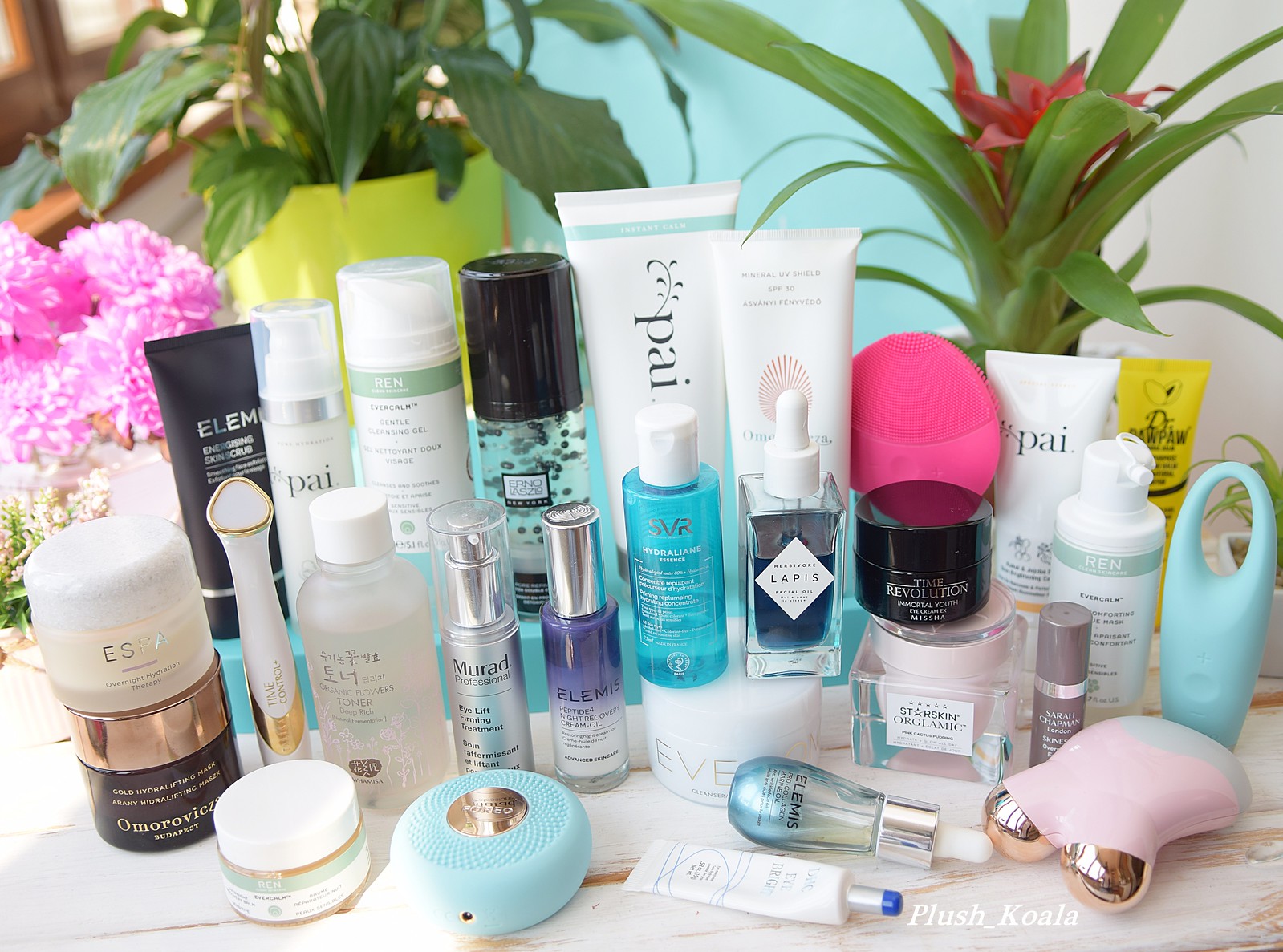A meticulously arranged collection of beauty products is displayed on a luxurious white marble table with distinctive brown marbling. The assortment comprises approximately 15 to 20 items, including various sizes of jars, bottles, and pump dispensers. Among these products is a notable pink and chrome massage device, featuring two chrome balls extending from the top. Most items are intended for eye, face, and skin care, with the majority capped in white and one distinctive spray can capped in black. 

In the backdrop, an aloe plant adds a touch of natural green, while several other potted plants of unknown species and a charming set of pink flowers are visible to the left. The arrangement suggests a meticulous and thoughtful layout, as if someone has carefully organized their extensive skincare collection for display.